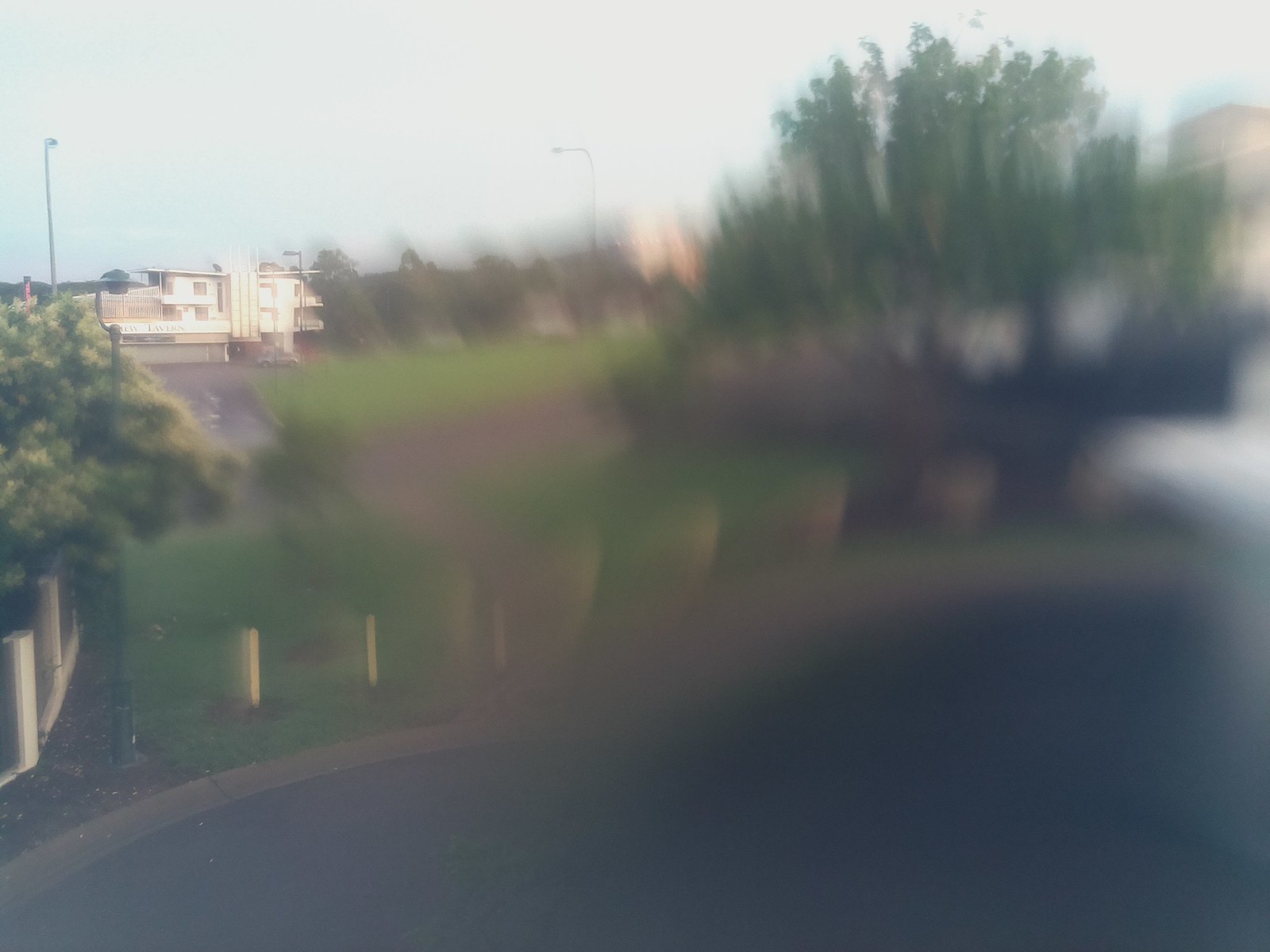In this heavily blurred photograph, a tree dominates the foreground, partially obscuring various details. Yellow stakes or poles line the grass along the curb, seemingly positioned to protect the yard from incoming vehicles. Beyond this, a patch of blacktop is visible, contributing to the urban setting. The midground reveals a white building with a flat roof, which could be an apartment complex or a hotel, given its balconies and the sign that reads, "Something View Tavern." A gray pickup truck is parked outside the building, and the blacktop driveway leads directly to it. The sky is a very pale blue, setting a muted backdrop. On the far right, there is a faint, ivory-colored structure that is difficult to discern due to the photograph's blurriness.